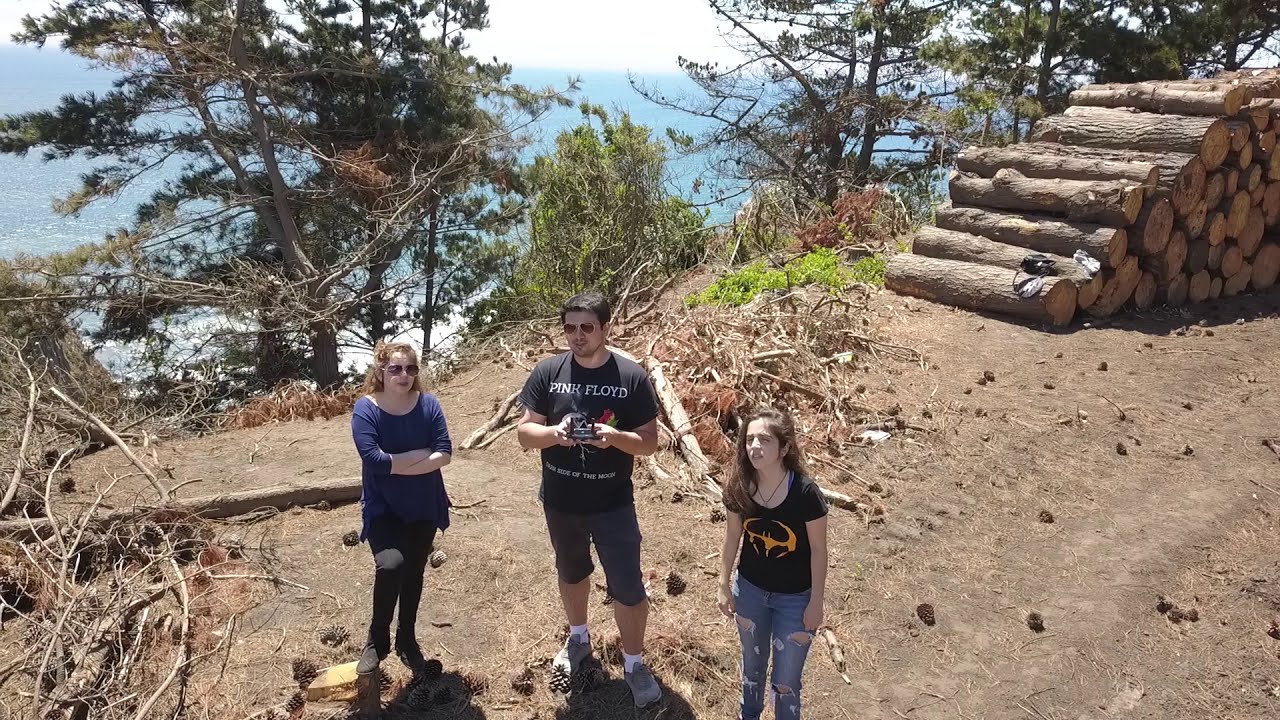The outdoor image, a color photograph in landscape orientation, captures a scenic moment involving three people standing on a dirt path in a wooded area, likely taken by a drone. The man in the middle, approximately six feet tall with short dark hair and wearing sunglasses, is dressed in a "Pink Floyd: Dark Side of the Moon" black t-shirt, knee-length shorts, and tennis shoes. He holds a remote controller, presumably for flying a drone, which they are all looking at. To his left stands a young woman, possibly a teenager, with long dark hair. She is dressed in a black t-shirt adorned with a gold and black design reminiscent of the Batman logo, paired with torn blue jeans and a necklace. On his right, an older woman, possibly their mother, has short dark hair and wears a blue long-sleeve tunic and black pants, her arms crossed and also donning sunglasses.

The background features a picturesque scene with green trees, cut and neatly stacked firewood to the top right, and what appears to be a body of water or an ocean further back, contributing to the serene ambiance. Pine cones are scattered across the ground, adding to the natural aesthetic of the wooded area. The composition and details suggest the image's style as photographic realism, captured from a high vantage point indicative of drone photography.